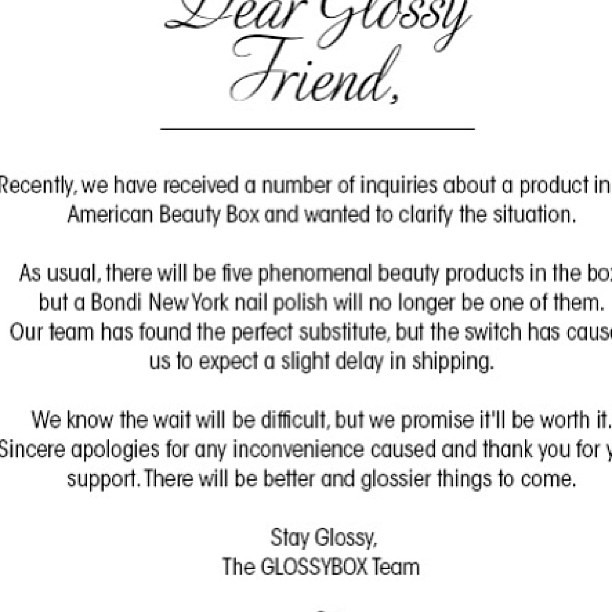The image depicts a formal letter from the American Beauty Box to its customers, presented as black text on a white background. The letter opens with "Dear Glossy Friend" written in cursive, followed by a line underneath. The body of the letter addresses recent inquiries regarding a product in the American Beauty Box, explaining that due to a discontinuation of the Bondi New York nail polish, the box will no longer include this item. However, a perfect substitute has been found, which will cause a slight delay in shipping. The letter assures customers that the wait will be worthwhile and apologizes for any inconvenience. It concludes with a hopeful note, stating, "There will be better and glossier things to come," and is signed off with "Stay Glossy, Your Glossybox Team." The entirety of the text is centrally aligned and occupies about a paragraph and a half in the middle of the page.